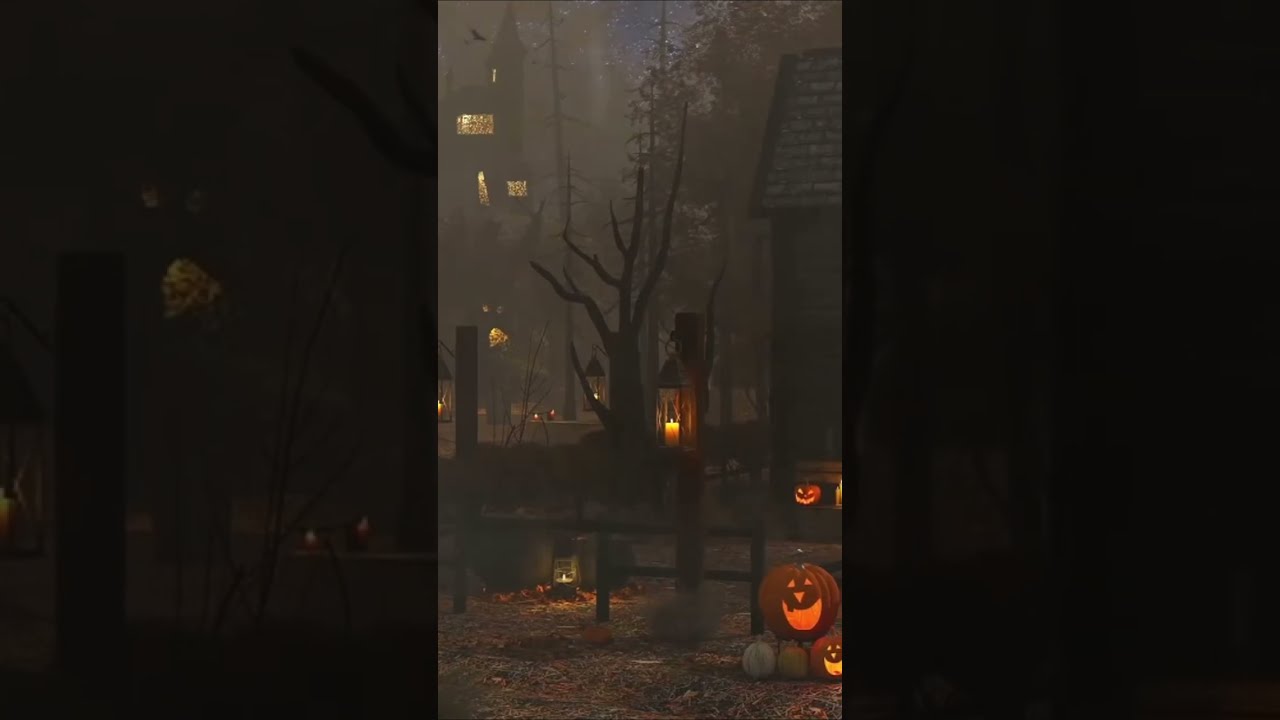The eerie Halloween scene in this dark, gothic image is set against the backdrop of a spooky neighborhood. In the foreground, a pair of jack-o'-lanterns, one large and one small, sit amidst a cluster of white pumpkins next to a weathered black fence with two tall posts—one of which supports an old-fashioned lantern. Leaves carpet the ground, enhancing the autumn atmosphere. A leafless tree, possibly artistically crafted for a haunted exhibit, holds another hanging lantern, casting an ominous glow. To the right, a portion of a quaint, Victorian-style house with lit windows is visible, hinting at a larger ghostly residence. A bench featuring another jack-o'-lantern is positioned nearby. The entire scene appears like a screen capture from a smartphone, capturing the chilling essence of Halloween night. In the distance, another illuminated house stands framed by both leafless and leaf-covered trees, adding layers of depth and mystery to the image.